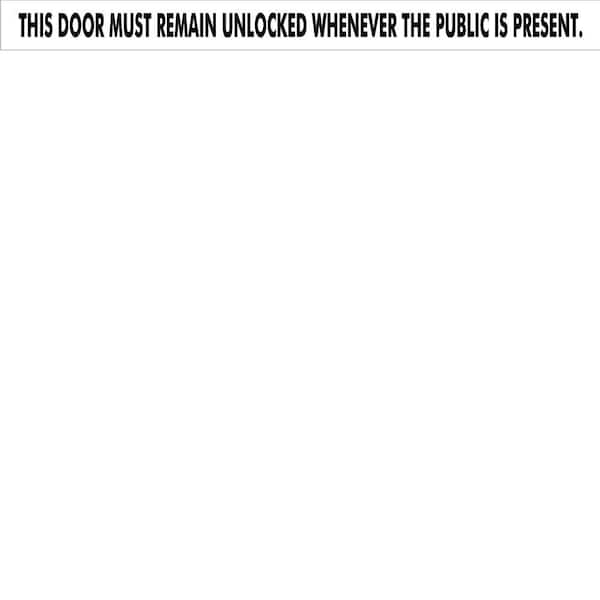The image is presented on a white canvas, with 90% of the canvas remaining blank and pristine. At the top of the image, a bold, black inscription declares, "This door must remain unlocked whenever the public is present, period." Directly beneath this directive, a thin gray line runs horizontally, serving as a subtle divider between the text and the empty expanse below. The remainder of the canvas is devoid of any additional text, characters, colors, or imagery, creating a stark, minimalist contrast to the prominent message at the top.